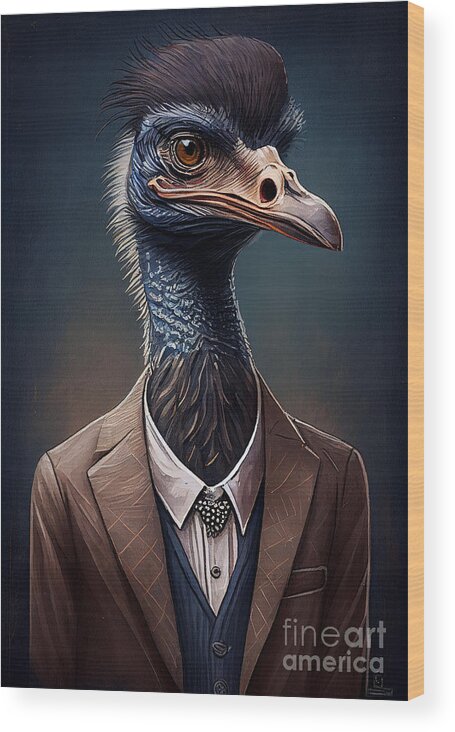The image depicts a digital painting from Fine Art America featuring a bird with dark blue feathers that resemble the head of an emu. The bird, characterized by its large beak and tan, hazel eyes, is portrayed in a sophisticated manner, dressed in a brown business suit. Beneath the suit is a blue button-down shirt, layered with a white collared shirt and accented with a black bow tie adorned with white spots. Its plumage includes tufted feathers on its head resembling hair and slight white feathers trailing behind its neck and head. The bird is shown from a front point of view with its head intriguingly tilted to the side, giving it an air of thoughtfulness. The background is predominantly dark blue with subtle touches of brown and orange accents. The artwork's lower right corner features a Fine Art America watermark in silvery text. The image appears to be a printed preview on a canvas with a wooden finish, slightly offset from the wall.